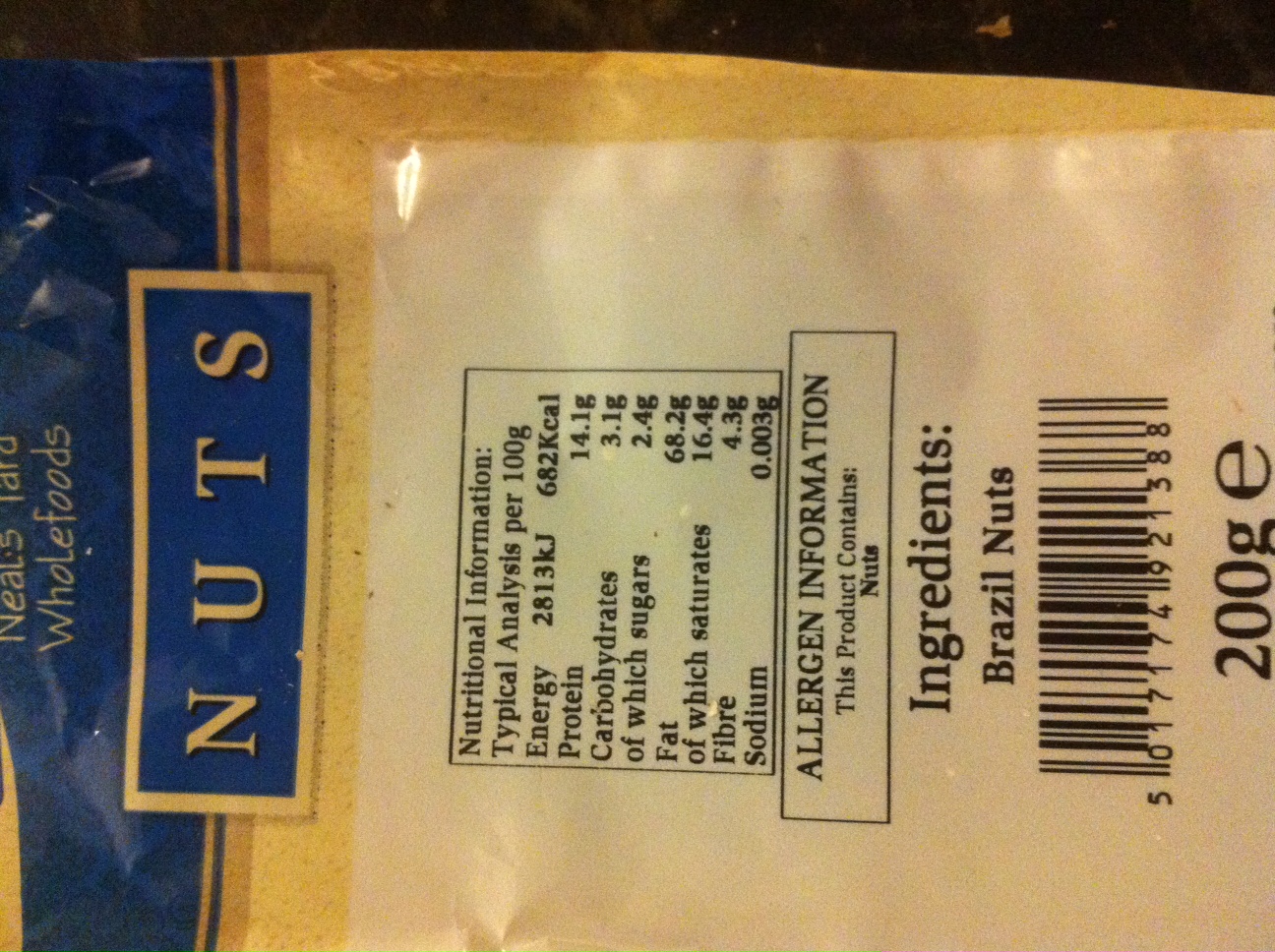The image depicts the back of a package of Whole Foods Brazil nuts. The top section of the package features a blue background with "Whole Foods Nuts" written in yellow letters. The central part of the image contains detailed nutritional information: energy 2813 kJ (682 kcal), protein 14.1 grams, carbohydrates 3.1 grams (of which sugars 2.4 grams), fat 68.2 grams (of which saturates 16.4 grams), fiber 4.3 grams, and sodium 0.003 grams. An allergen notice clarifies that the product contains nuts, specifically Brazil nuts, listed as the ingredients. At the bottom of the package is a UPC code, essential for scanning at checkout, and the total weight of the nuts, which is 200 grams.